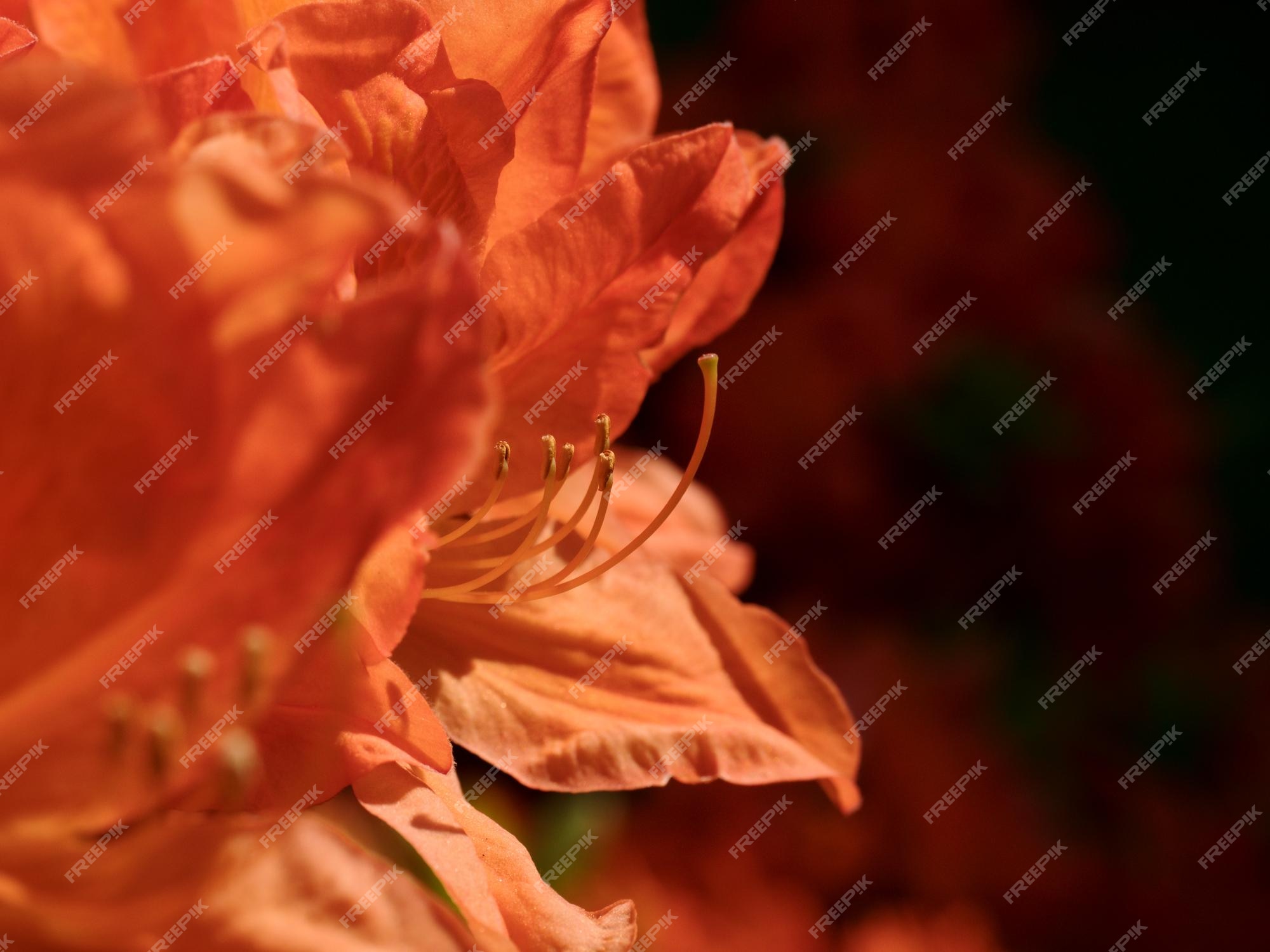The image is a close-up of a vibrant peach-colored orchid with various shades of peach and some rosy pink hues. It showcases the flower's numerous, slightly wrinkled petals, which appear almost silk-like. Prominent among the petals are the pollen pods, displaying a pink hue with gold-colored tips. The orchid’s bulbs or sepals are visible, extending from the top. The background is a rich mosaic of dark maroon, black, and patches of green and yellow, though it is deliberately blurred to accentuate the flower. Overlaid throughout the photograph is a watermark that reads "Freepik" in a column and row format, subtly filling the negative space. The orchid is beautifully illuminated, making its colors exceptionally vibrant against the darker, subdued background.